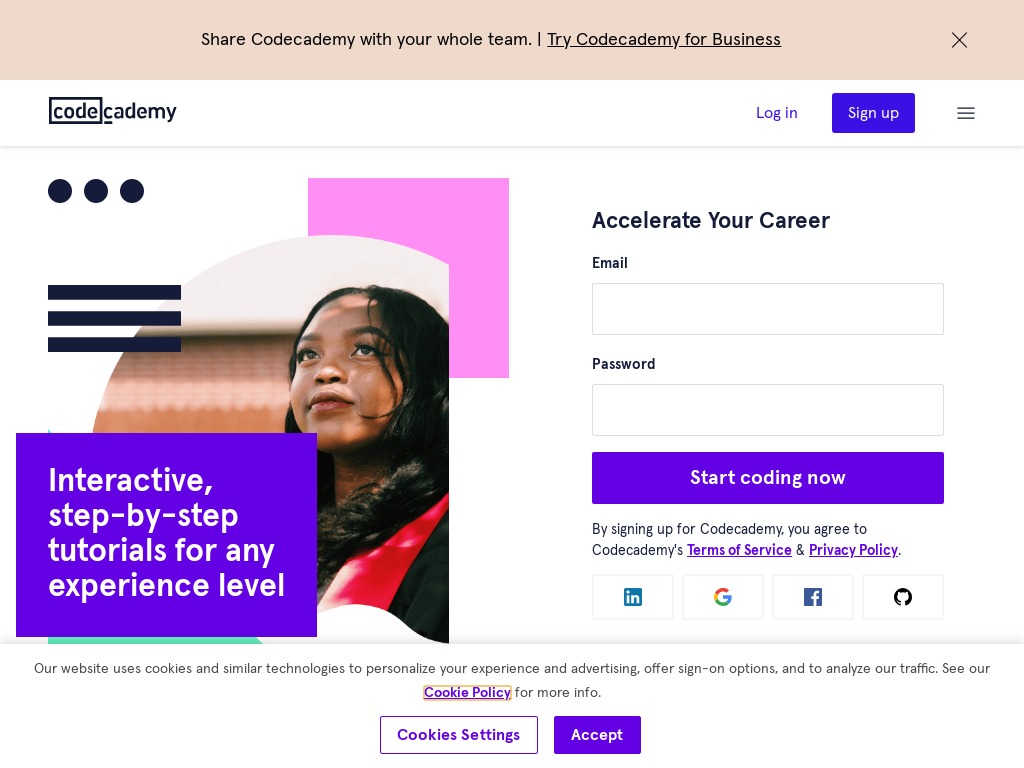Screenshot Description:

The provided image is a detailed screenshot from a webpage. The top section of the screenshot features a tan-colored stripe running from the upper left to the upper right. Within this stripe, centered text reads "Share Code Academy with your whole team. Try Code Academy for business," which is underlined, indicating it is a live link. On the far right of this stripe, there is an 'X' icon for closing the banner.

Below this stripe, the company's logo "Codecademy" is prominently displayed on the left side of the header. To the right of the logo, there are three elements: a live link labeled "Login," a blue "Sign Up" button, and a menu icon consisting of three horizontal lines.

A light gray horizontal line spans from left to right under the header. The main body of the page is divided into two columns. The left column consists of an illustrative image, while the right column hosts a user sign-up form.

In the form on the right, the headline "Accelerate your career" is displayed. Below this, there are fields for the user to enter their email and password. The fields are followed by a large blue button with the text "Start Coding Now" in small font.

The background of this section is blue. Under the form, there is a statement reading, "By signing up for Codecademy, you agree to Codecademy's Terms of Service" and "Privacy Policy," both of which are live links highlighted in purple.

Further down, social media icons for LinkedIn, Google, and Facebook are shown, along with one unrecognized icon. Below these icons, a notice about the "Cookie Policy" is encased in an orange outline, possibly drawn by someone.

Lastly, there are two buttons at the bottom for cookie preferences: "Cookie Settings" on the left and "Accept" on the right. The "Accept" button is purple while the "Cookie Settings" button is blue.